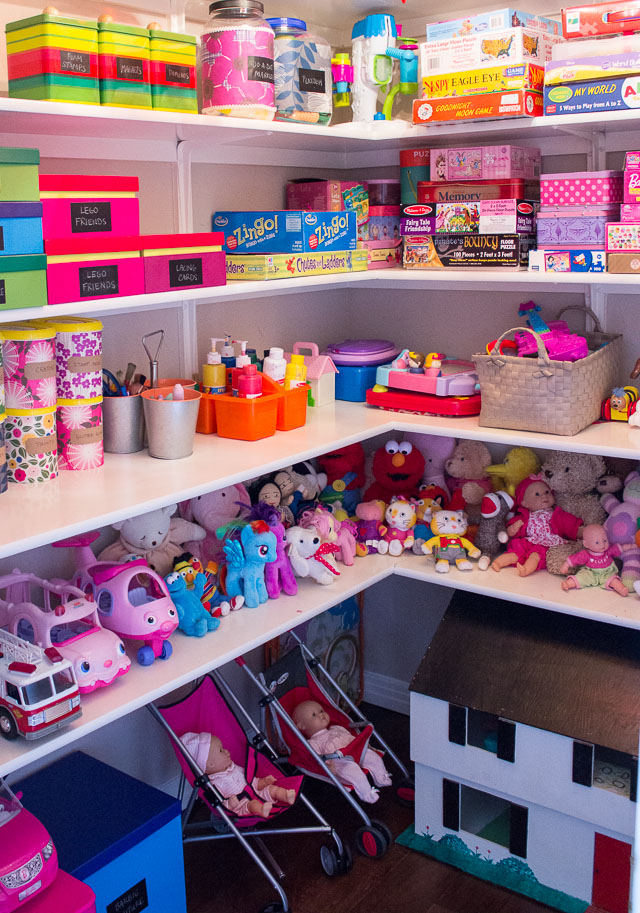The image depicts a cozy corner of a shop that resembles a daycare or children's play area, showcasing a neatly organized array of children's toys and essentials. The scene is framed by white, L-shaped shelves that extend vertically across the wall, filled with vibrant and playful items. 

On the bottom shelf, there is a charming assortment of stuffed animals, including beloved characters like Cookie Monster, Bert, Ernie, and My Little Ponies. Nearby, toy vehicles such as fire trucks add to the whimsical display. Directly above, the second shelf houses a basket with small toys, an orange bin brimming with paint bottles, and various cylindrical canisters with colorful labeling. 

Ascending to the third shelf, there are cardboard boxes likely containing board games like Zingo and Chutes and Ladders, alongside metal tins filled with markers and other art supplies. The topmost shelf features more cardboard boxes and jars, contributing to the delightful clutter. 

The floor beneath the shelves is wooden and brown, grounding the vibrant shelves above. Here, baby strollers and a quaint dollhouse, complete with a brown roof, add an additional layer of charm and utility to this vibrant, child-friendly nook.